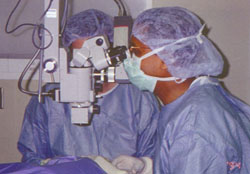The photograph depicts two medical professionals, likely surgeons, engaged in a procedure in a clinical setting. Both are wearing light blue surgical scrubs, including full face masks and somewhat translucent blue hairnets. The scene captures them operating on a patient partially covered with a purple and white surgical drape. The surgeon on the left, identified as a white male with glasses, is intently looking through an advanced electronic magnifying device or microscope mounted above them. This device has a lens directed downwards, several wires hanging from its sides, and appears to aid in magnification during the procedure. The second person, partially obscured by the microscope, is similarly dressed but their gender is indeterminate from the image. The clinical background is an off-white color, contributing to the stark and sterile environment of the operating room.